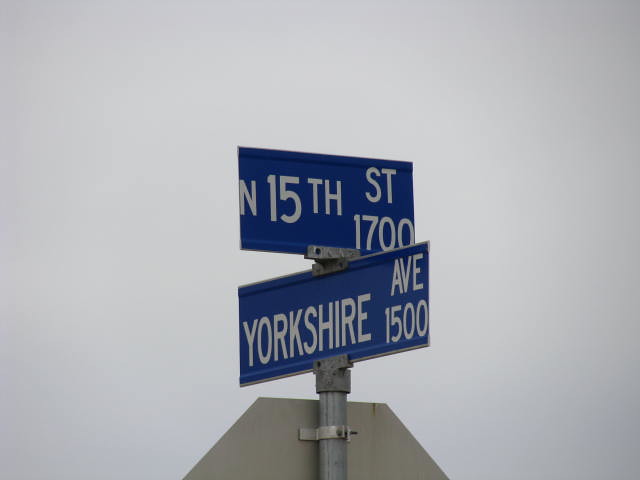The image shows a series of three signs mounted on a pole against a white, likely cloudy, background. The topmost sign reads "N 15th Street, 1700," denoted with white letters on a blue background. Below it, the middle sign states "Yorkshire Avenue, 1500," also featuring white letters on a blue background. The third sign, positioned at the bottom, is visible only from the back, making its text unreadable from the image's perspective. The white background suggests an overcast sky, giving the scene a monochromatic and somewhat muted atmosphere.